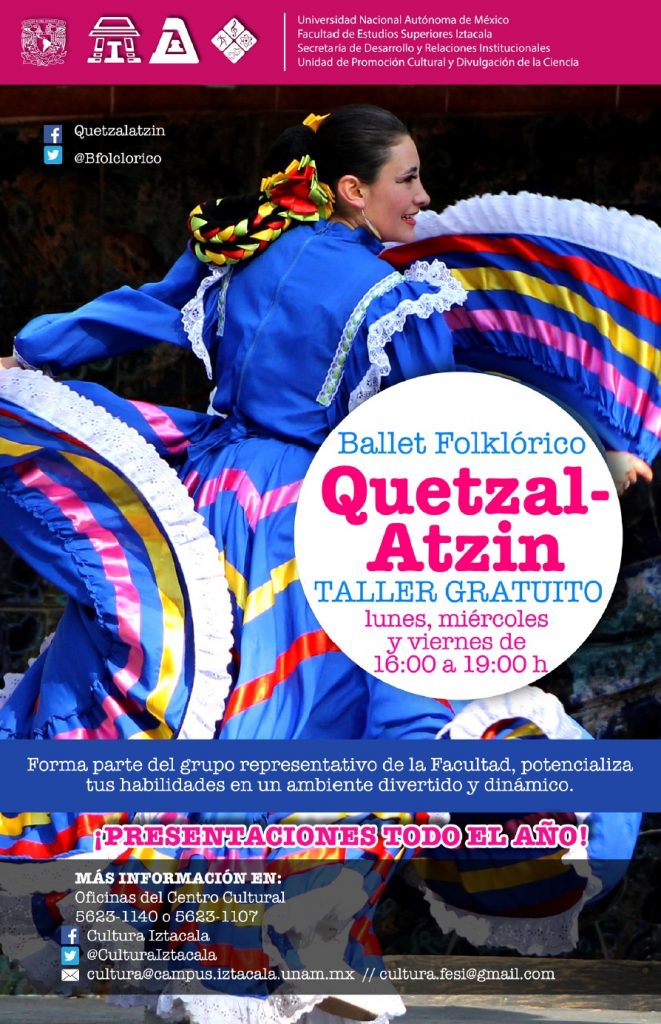The image depicts a vibrant and eye-catching social media flyer in Spanish, featuring a woman in motion, spinning gracefully in an elaborate, long, flowy gown predominantly blue with white edges and adorned with zigzag lines in pink, yellow, and red. The woman, likely a performer, is captured in a dynamic side profile pose, facing towards the right. The flyer prominently displays the text "Ballet Folklórico" within a white circle and mentions "Quetzalatzin" and "Tour Gratuito" in pink. The background includes additional graphic elements such as colored rectangles with unreadable white text, and social media icons for Twitter, Facebook, and email, suggesting it's designed to promote an event or performance, possibly related to South American or Mexican cultural heritage. The overall color palette includes light pink, black, blue, yellow, red, light purple, and orange.